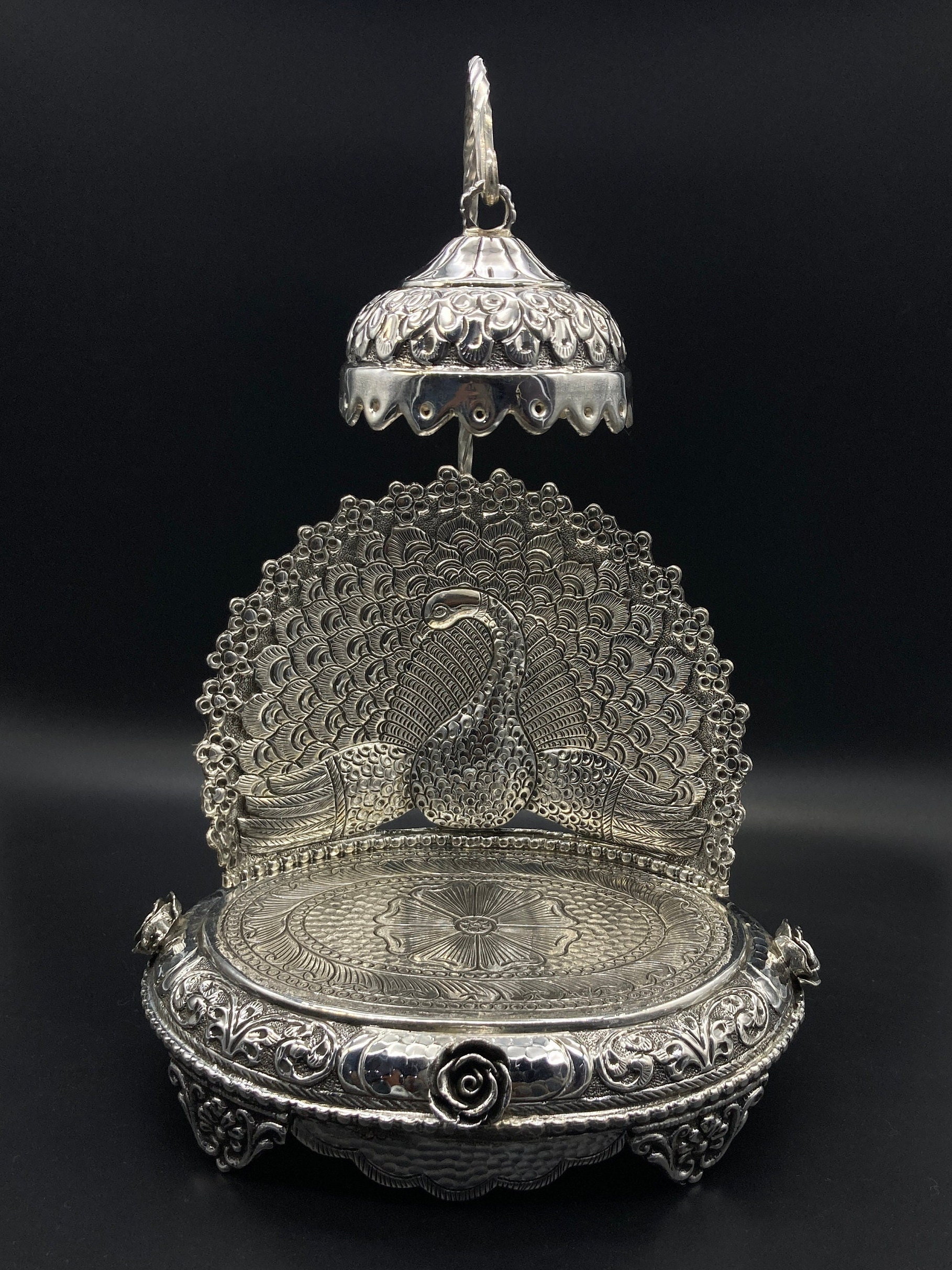This is a close-up photograph of an intricately designed antique object set against a black background, illuminated by a whitish light from above. The item is made of a gleaming silver metal, and it features a circular, highly ornate base adorned with three curved decorations resembling rose petals, each situated evenly around the circumference. The base is supported by triangular, ornate legs.

Rising from the back of the base is an elegant U-shaped structure that may depict a bird, possibly a swan or peacock, with detailed feathers or engravings adding to its graceful appearance. From the top of this U-shaped frame extends a curved metal pole, from which a small cap-like lamp hangs, casting light over the centerpiece. The overall design is notably unique and ornate, with a harmonious blend of artistic elements that suggest it could be a brooch or a similarly decorative item, though its exact function remains unclear.